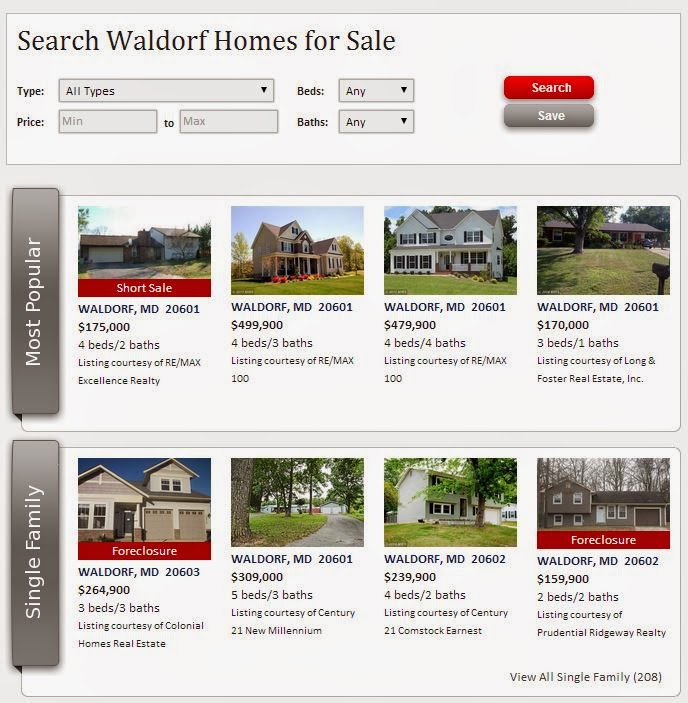**Detailed Caption:**

The image is a screenshot of an online real estate search interface for homes for sale in Waldorf. At the top of the screen, there is a white search bar with the header "Search Waldorf Homes for Sale." Within this search bar, there is placeholder text that says "Type all types," accompanied by a drop-down menu. Below the main search bar, there are two narrower text boxes for price input, labeled "Minimum" and "Maximum." To the right of these text boxes, there is another drop-down menu for selecting the number of beds, which currently displays "Any." Adjacent to this is another drop-down for selecting the number of baths, which also displays "Any."

To the right of the drop-down menus, there is a prominent red search button with white text indicating "Search" and a gray button labeled "Save," also with white text. 

Below this main search interface, the content is divided into two sections. The first section is titled "Most Popular," showcasing various Waldorf homes:

1. A short sale property in Waldorf, MD 20601 listed at $175,000, featuring 4 beds and 2 baths.
2. A home priced at $499,900 with 4 beds and 3 baths.
3. Another property priced at $479,900, offering 4 beds and 4 baths.
4. A more affordable home listed at $170,000, which includes 3 beds and 1 bath.

The second section is titled "Single Family" and lists:

1. A foreclosure property in Waldorf, MD 20603, priced at $264,900, with 3 beds and 3 baths.
2. A home listed at $309,000, featuring 5 beds and 3 baths.
3. Another listing at $239,900 with 4 beds and 2 baths.
4. The final property in this section is another foreclosure, priced at $159,900, offering 2 beds and 2 baths.

The layout of the webpage emphasizes ease of comparison between different properties through concise summaries and clear organization.